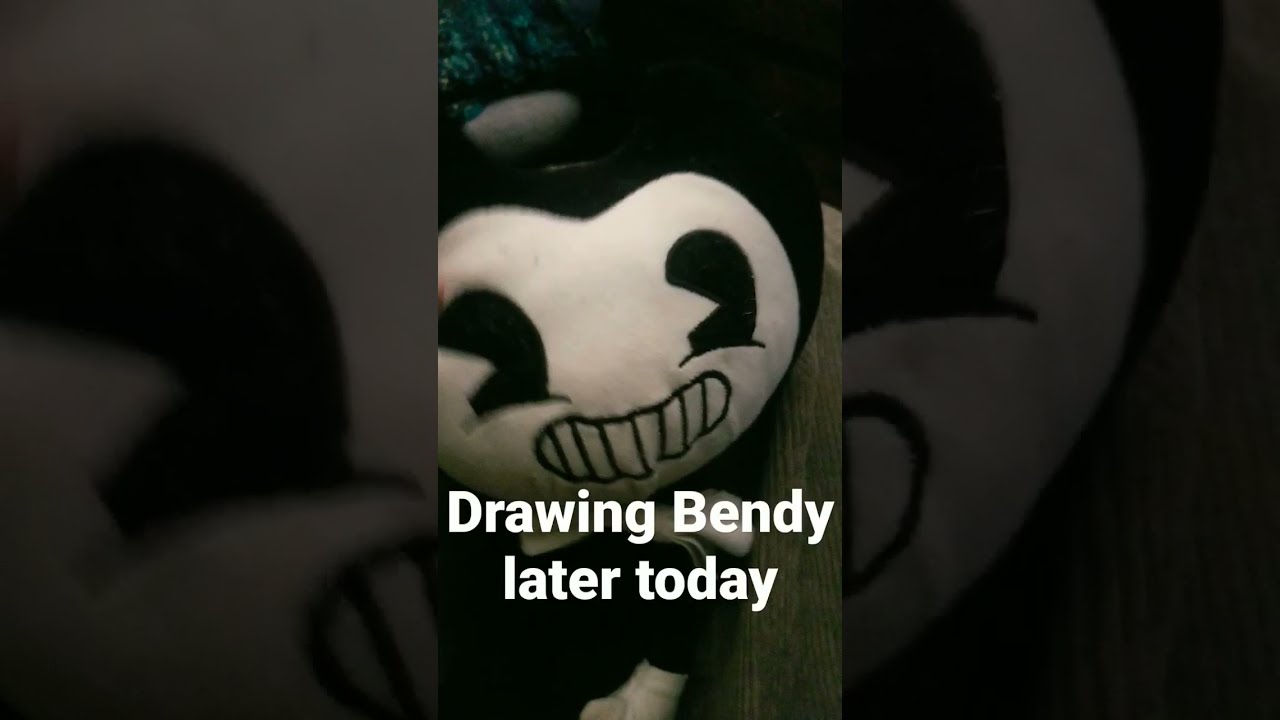The image features a stuffed toy, specifically Bendy from the video game "Bendy and the Ink Machine." Bendy has a crescent-shaped black head, a heart-shaped face, pie-cut black eyes, and a toothy grin. His black body is adorned with white gloves and a white bow tie. The toy's large face takes up much of the image, which has been edited with a dark filter and blown up, creating an out-of-focus border that frames the central figure. The toy appears to be placed sideways, with the ground to its right and some indistinct bluish and whitish shapes in the upper left. Overlaying the image, in white text, are the words "Drawing Bendy Later Today." The text and the enlarged, darkened background add an interesting contrast, making the cheerful yet eerie face of Bendy the focal point.